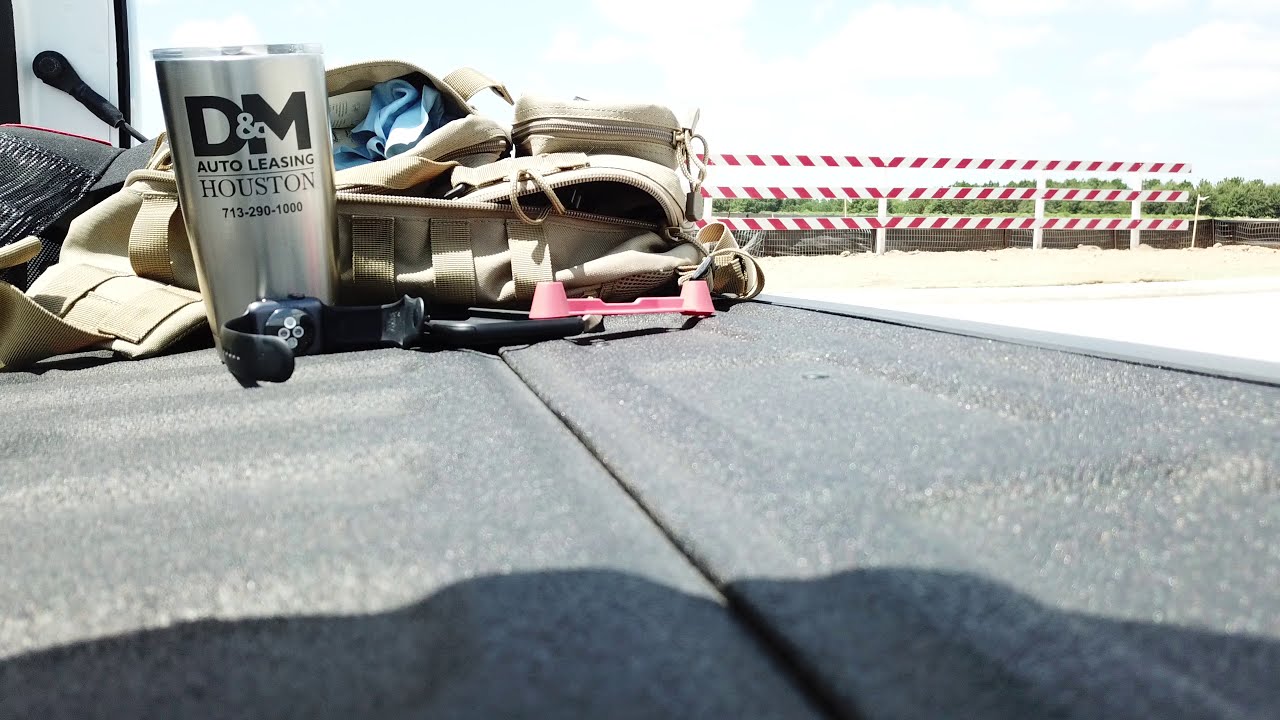This is a low-angle shot taken from what appears to be the flatbed of a truck, with the camera likely resting on the textured surface. A gray backpack with noticeable straps lies in the foreground, accompanied by a metal coffee cup marked "DNM Auto Leasing Houston 713-290-1000" and an Apple Watch. There is also a tool belt and a baseball cap next to the backpack. Not far from this setup, a distinctive white and red barrier, resembling a dead-end or do-not-enter sign, extends horizontally with three boards. The truck appears to be parked at the roadside, with some vegetation and possible fruit trees or an orchard visible in the background, suggesting a rural setting. The sky above is overcast and white, adding to the scene's subdued atmosphere, perhaps indicating that this is a preparatory setup for some kind of outdoor photography project.